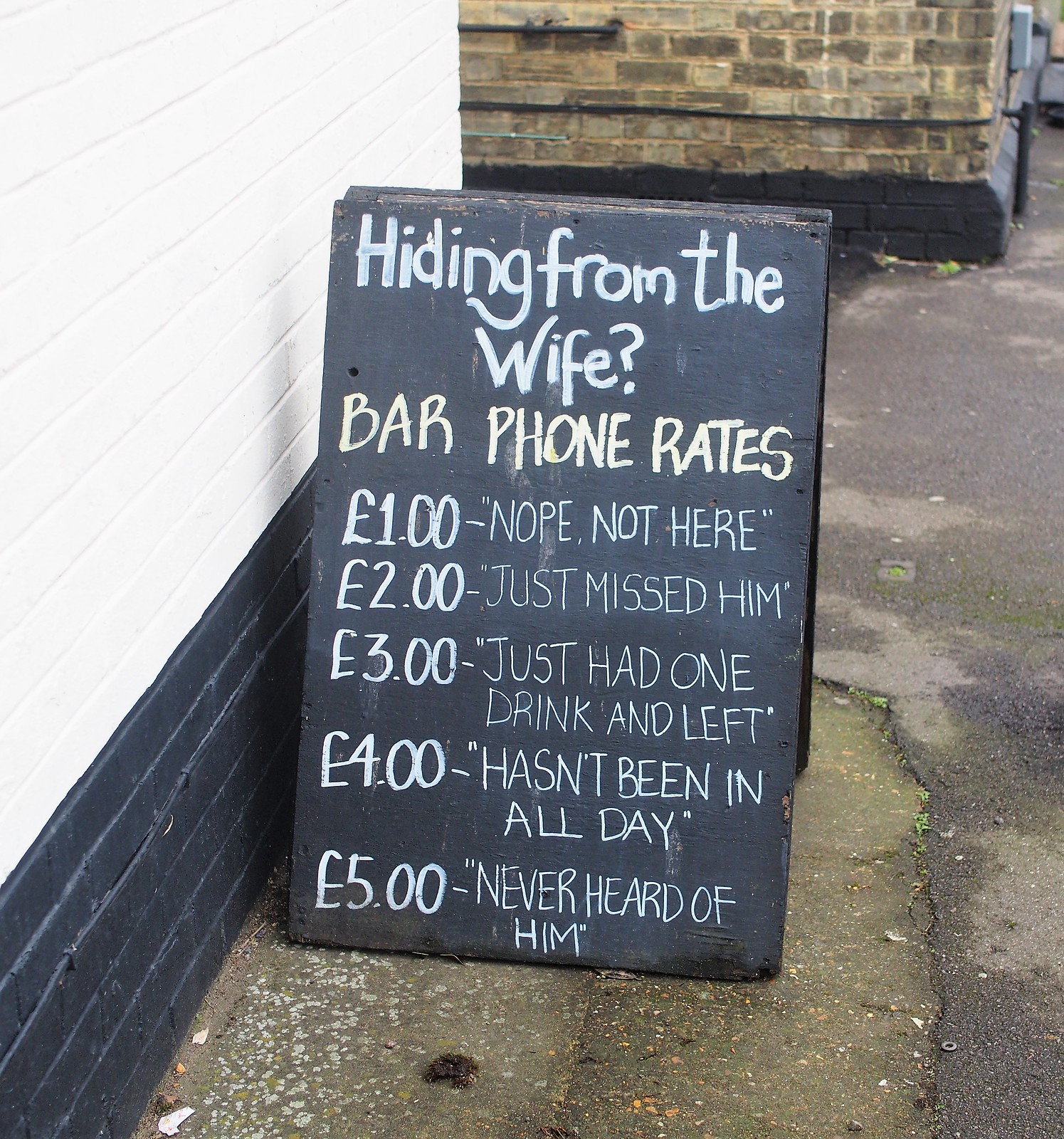In this detailed close-up image, a triangular sandwich board sign is prominently displayed on a slightly recessed, brown pavement, distinct from the surrounding gray pavement. The sign is propped up and positioned against a brick wall with two-tone paint: white on the upper part and blue on the lower part. The main text on the sign, written in white and off-white letters, humorously details escalating bar phone rates associated with various excuses for a man's whereabouts, titled "Hiding from the wife." The exact rates and messages are as follows: "1 pound - Nope, not here," "2 pounds - Just missed him," "3 pounds - Just had one drink and left," "4 pounds - Hasn't been in all day," and "5 pounds - Never heard of him." In the background, another brick wall is seen, painted brown at the top and black at the bottom, complete with a black pipe standing adjacent. To the left of the sign, another building's façade is visible, with its upper half painted white and the lower half painted black.